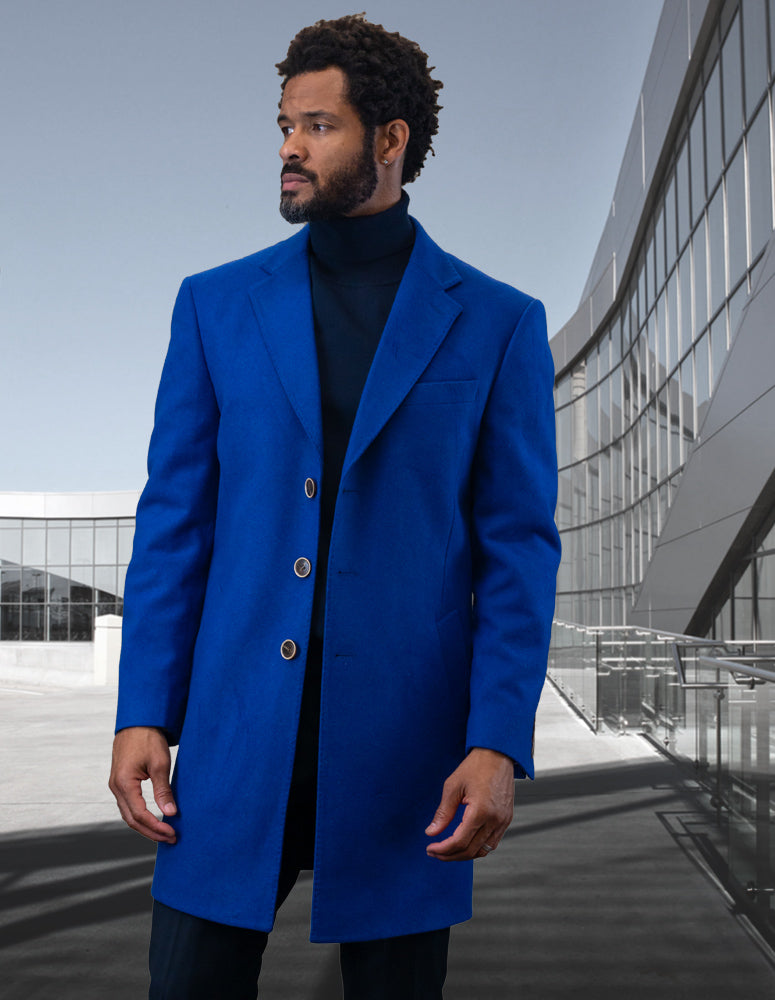In this detailed photograph, a handsome brown-skinned black gentleman with a medium build and a full beard and mustache stands confidently, gazing off into the distance to his left. He is adorned in a stylish dark blue wool three-button overcoat, complemented by a black turtleneck and black pants. His natural, medium-length, slightly curly afro adds to his striking appearance, accentuated by a subtle earring that glints in the daylight. Behind him, a contemporary glass building with an intricate structure of windows and metal barriers rises from low to high, featuring grey and white stone elements along its base. The glass building, bathed in sunlight against a greyish sky, enhances the modern, architectural elegance of the scene, hinting at a concrete flooring within this sophisticated outdoor setting. The man’s model-like poise against this sleek, urban backdrop creates a visually compelling image of refined style and presence.